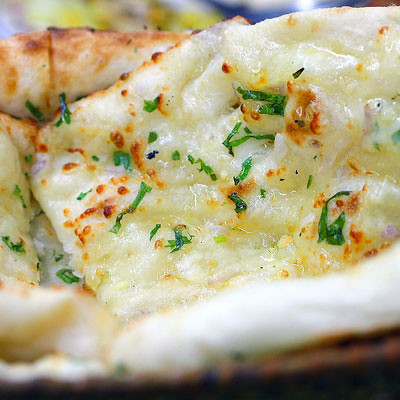This close-up color photograph showcases a plate of cheesy bread (or pizza) that fills nearly the entire square frame, leaving only a blurred hint of the background. The golden, melted cheese is speckled with green herbs, likely parsley or basil, and exhibits enticing brown toasty spots, indicating the cheese has been baked to a delectable finish. The foreground prominently features the white crust, which is also toasted, with some slightly blackened, crispy edges where it might have been overdone, enhancing its crispy texture. The bread appears somewhat greasy and is sliced, but the pieces are so closely stacked that individual slices are difficult to distinguish. The base of the brown plate is just visible at the bottom of the image. Overall, the detailed texture and color make this cheesy bread look incredibly delicious and appetizing.